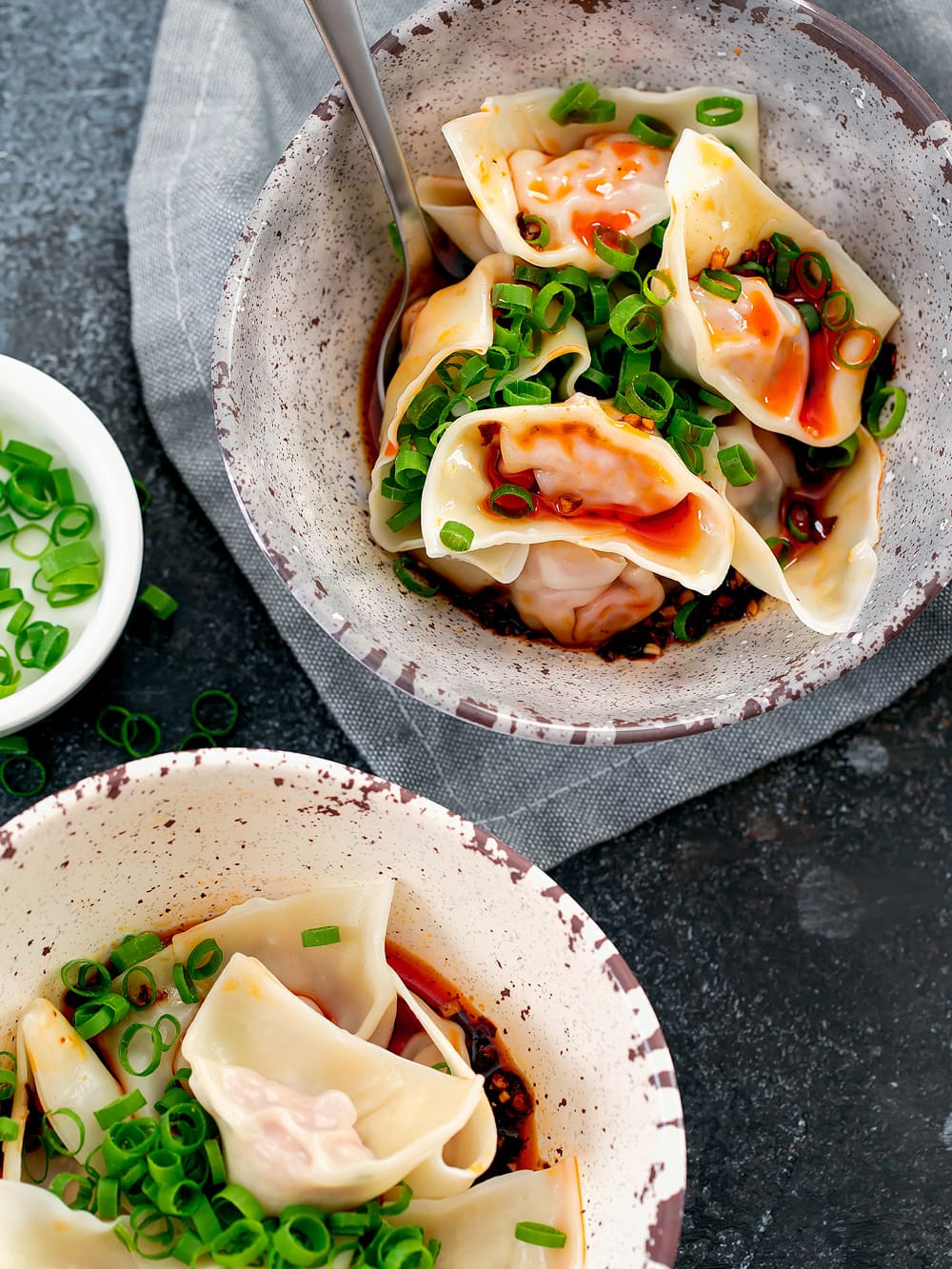The photograph captures an overhead view of a dining scene, possibly set outdoors at a picnic or indoors on a gray tabletop. In the lower left section of the image, a white plate with brown markings is filled with dumplings in a vibrant red broth, accompanied by a generous amount of scallions. The top right of the image reveals a matching beige or off-white bowl with brown markings, containing three open dumplings showing shrimp filling, nestled among more scallions, and a silver spoon. Partially visible between the two dishes is a small bowl of additional scallions. The setting is free of any text, focusing solely on the enticing array of food presented on a neutral gray surface. The colors in the image range from the red of the broth to the green of the scallions, the tan and white of the dumplings, and the slate gray of the tabletop, creating a harmonious and appetizing scene.